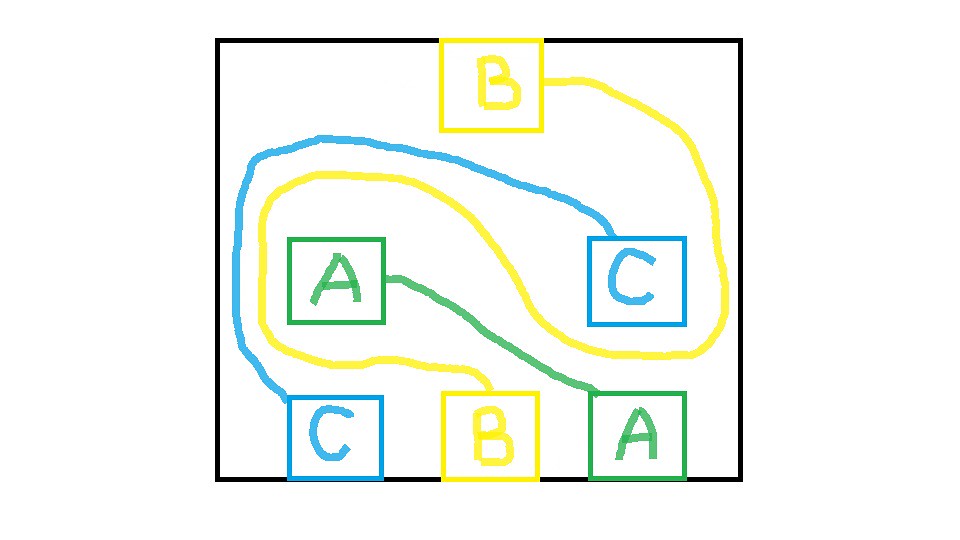In the image, each letter (A, B, and C) is enclosed within its own box, and lines connect corresponding letters without intersecting. The A's are marked in green, the B's in yellow, and the C's in blue. The layout of the boxes is as follows:

- The top row has a solitary B.
- The middle row contains an A on the left and a C on the right.
- The bottom row houses a C, a B, and an A, from left to right respectively.

Each letter has a corresponding colored line connecting it to another box with the same letter. The connections are detailed as follows:

- The yellow line from the B at the top goes from the B downwards, navigating between the green and blue lines for A and C without intersecting them, reaching the B at the bottom.
- The green lines from the A's are direct, connecting corresponding A boxes straightforwardly.
- The blue lines for the C's curve around the yellow line associated with the B's to connect their respective boxes without any lines crossing.

This meticulous arrangement ensures that each line remains distinct and unconnected from other lines, creating a clear and organized visual relationship between the letters.